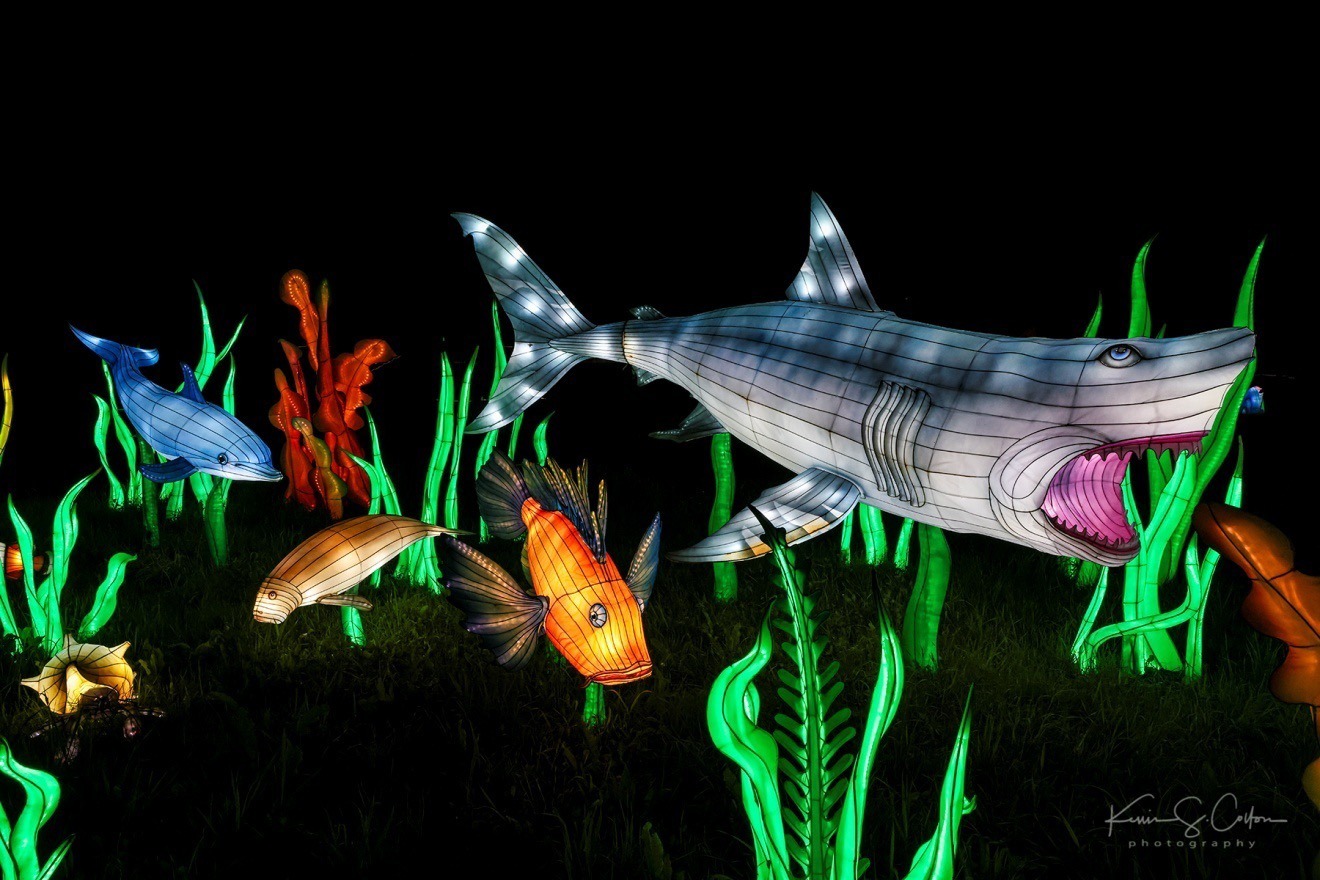The image features a vibrant and stylized neon art installation against a black background, reminiscent of gazing into an aquarium. The scene is illuminated by internal lights within the various ocean creatures, giving them a 3D appearance. In the center, there is an orange lionfish with brown fins. To the top right, there is a large hammerhead shark with a wide-open mouth, displaying a gradient of dark gray on top and light gray on the bottom. The top left corner showcases a small blue dolphin with a white chin, facing right, and below it is a brown manatee-like creature facing left. Among the bright and neon green, flowing aquatic plants that resemble blades of grass, there's also vibrant coral in shades of green and orange. Additionally, visible in the image is the name "Kimberly" followed by an illegible last name in the bottom right corner. The entire scene creates a vivid and fantastical undersea world.